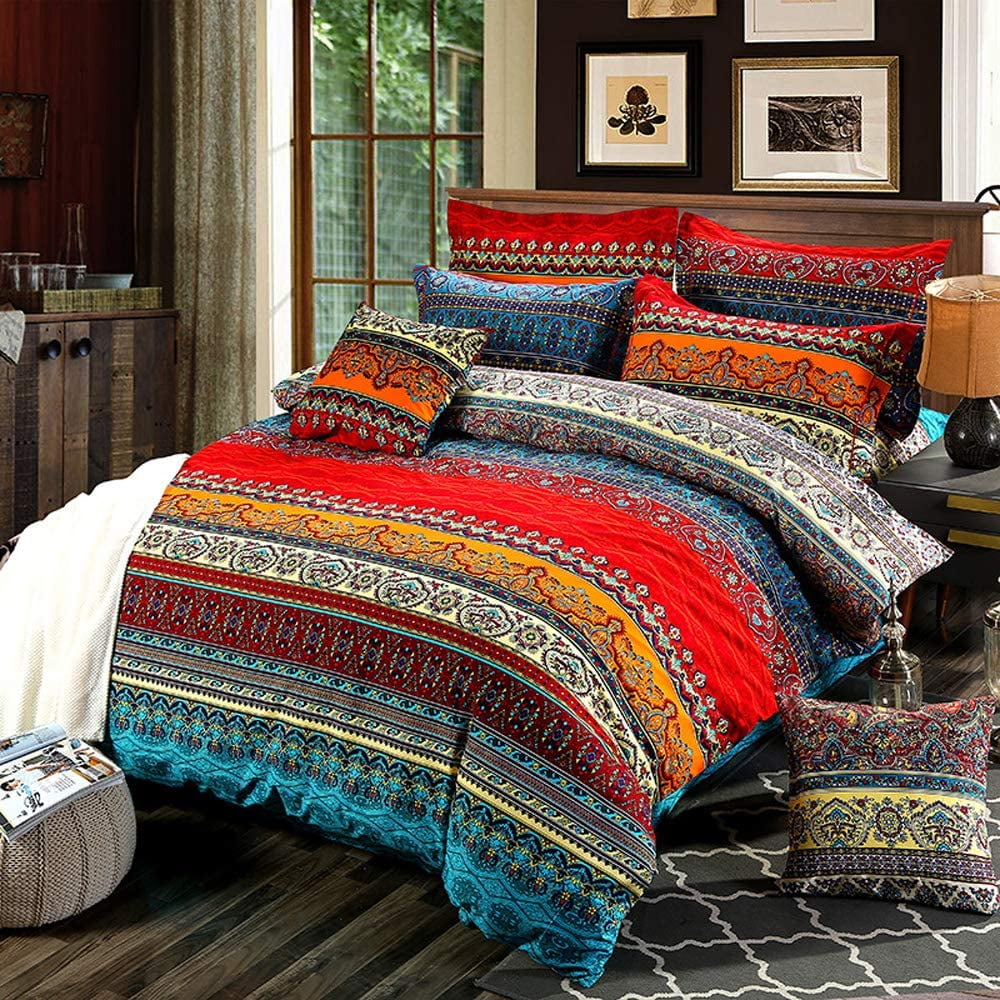This interior photograph of a bedroom features a centrally positioned bed adorned with a vibrant, multicolored duvet, exhibiting a rich array of stripes and complex patterns in hues of blue, yellow, red, black, orange, and gray. The bed is framed by an ornate wooden headboard and topped with five pillows: two large, two medium, and one small square pillow in the middle. Additionally, a similar multicolored pillow rests on the dark, almost black, hardwood floor beside a black and white patterned rug, lying adjacent to the bed. The walls are painted black with white wainscoting, and above the headboard, four framed pictures are displayed. To the right of the bed stands a nightstand with a dark-colored lamp. A glimpse of a potential glass door with curtains and what appears to be a wooden cupboard is seen on the left. The overall ambiance is an eclectic mix of old and new, with its ornate headboard and contemporary pop of colors on the bedspread.